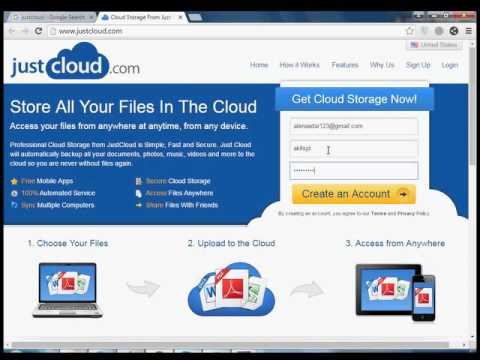This image captures a screenshot of the JustCloud.com website displayed on an internet browser with two tabs open. The active tab showcases the JustCloud.com webpage. The webpage features a predominantly white background with blue accents, presenting information on the advantages of using JustCloud for cloud storage. At the top right, there is a form where users can create an account by entering their email and password, facilitating easy access to cloud storage.

The central section of the webpage outlines a step-by-step guide to storing files in the cloud. The first step, depicted with an image of a laptop, instructs users to choose their files. The subsequent step, illustrated with files within a blue cloud, involves uploading these files to the cloud. Finally, the rightmost image shows various mobile devices, indicating the accessibility of the stored files across different platforms and devices.